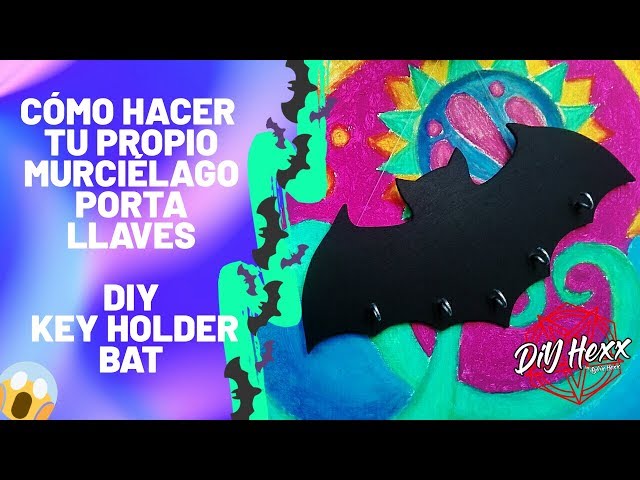This vibrant and playful advertisement features a DIY bat-shaped key holder with multiple hooks. The main focus is a large bat positioned centrally against a dynamic background that appears to be colored with crayon, blending shades of greens, blues, and purples. The left side of the background showcases muted tones of purple and pink with a tie-dye effect, while the right side bursts with varied and bright colors, reminiscent of childlike doodles.

In bold, uppercase white letters at the top left, the Spanish text "C-O-M-O H-A-C-E-R T-U P-R-O-P-I-O M-U-R-C-I-E-L-A-G-O P-O-R-T-A L-L-A-V-E-S" spells out instructions for making your own bat key holder. Below this, in English, it reads "DIY Key Holder Bat." Further down on the bottom right, the brand name "DIY HEXX" is elegantly inscribed in a slightly cursive white font. Adding a touch of whimsy, a gasping emoji with hands on its head is located at the bottom left, augmenting the surprise and delight evoked by the creative and functional key holder.